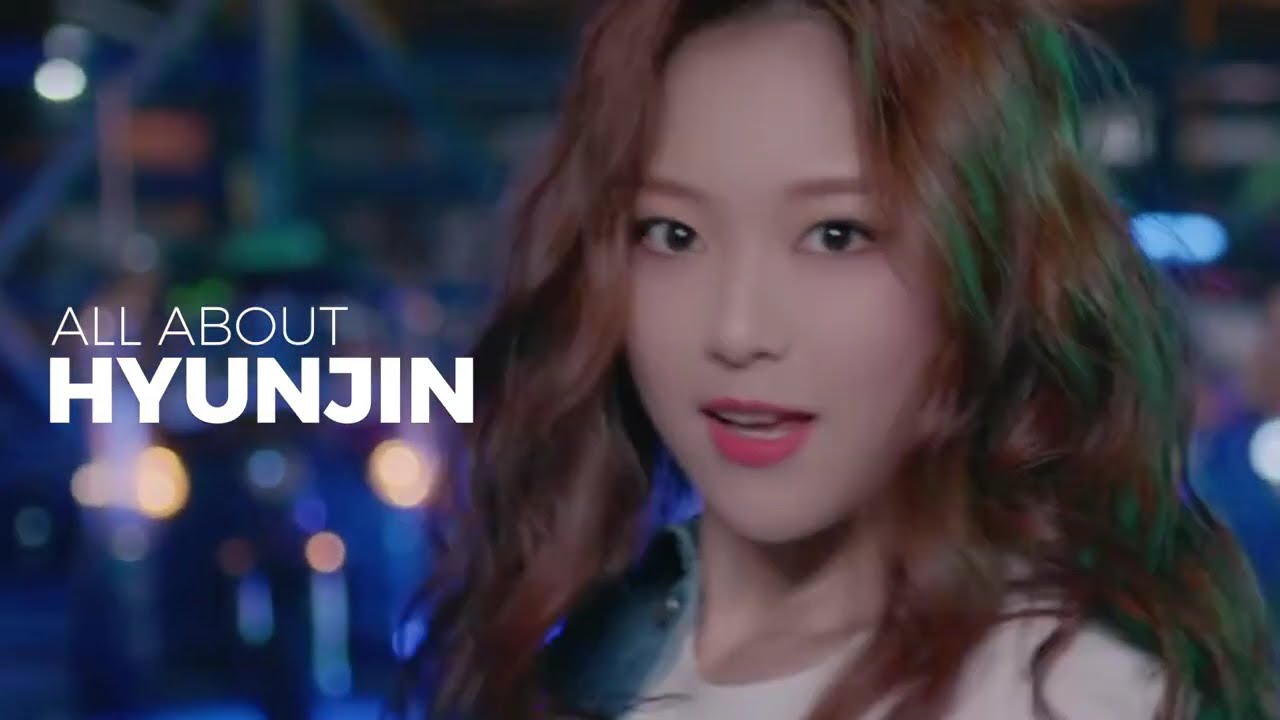The image appears to be a slightly blurry, close-up screenshot of an Asian woman, likely an actress or K-pop star named Hyunjin, turning towards the camera. She seems to be in motion, possibly singing or dancing, with long brown hair partially obscuring her face, styled with pink lipstick and holding a light skin tone. She faces us from a left-side profile with her gaze looking back over her left shoulder. The setting gives off a modern, dynamic atmosphere, possibly from a music video, live performance, or indoor show, accentuated by a background awash with blurred blue, white, and yellow lights reminiscent of electronic equipment or a nightclub scene. The text "all about Hyunjin," written in white font, is prominently displayed on the left side of the image, highlighting the focus on her. The overall image composition evokes a vibrant, contemporary aesthetic typical of K-pop visuals.